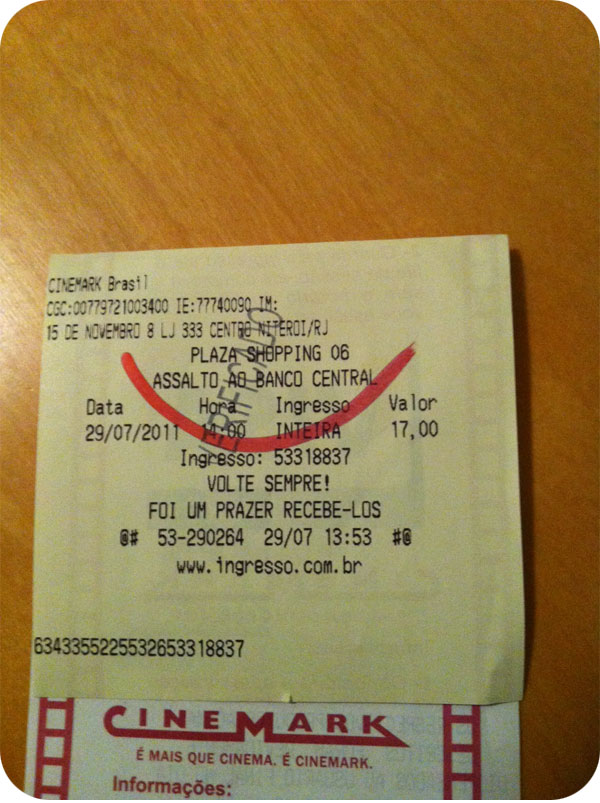This is a detailed description of a photograph featuring a cinematic receipt, predominantly from the Cinemark theater chain. The receipt itself is yellow and displays numerous numbers and codes in an indecipherable language, presumed to be either Portuguese or Italian. Prominently, the striking red Cinemark logo, familiar from various countries including the U.S., spans across the receipt with its stylized design featuring connected letters. The receipt indicates a date of the 15th of November and a location at Plaza Shopping, Salto a Banco Central. A URL, www.ingresso.com.br, is visible at the bottom, linking to a ticketing service, suggesting the theater's connection to Cinemark Brazil. The amount paid for the movie ticket appears to be 17 euros. Adding a touch of whimsy, a large red smile is hand-drawn across the receipt, and the word "Verificato," meaning "verified," is stamped vertically, confirming the transaction's completion. The receipt rests on a brown wooden tabletop.